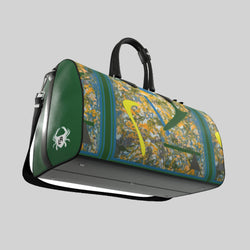This image features a vibrant and intricately designed duffel bag that appears to be levitating against a gray background, as its left side tilts upwards giving the illusion of motion. The bag features a solid black bottom and a black shoulder strap as well as two black handles on the top. The ends of the bag are a distinct forest green color, enhancing its striking appearance. The main body of the bag showcases a beautiful, abstract watercolor-like design with pastel colors, including green and blue stripes, and various splashes of yellow, orange, and white. This design is reminiscent of a fine piece of art, making the bag look like a canvas brought to life. Additional details include the black leather components and a potential subtle illustration or logo, adding to its luxurious and unique aesthetic.